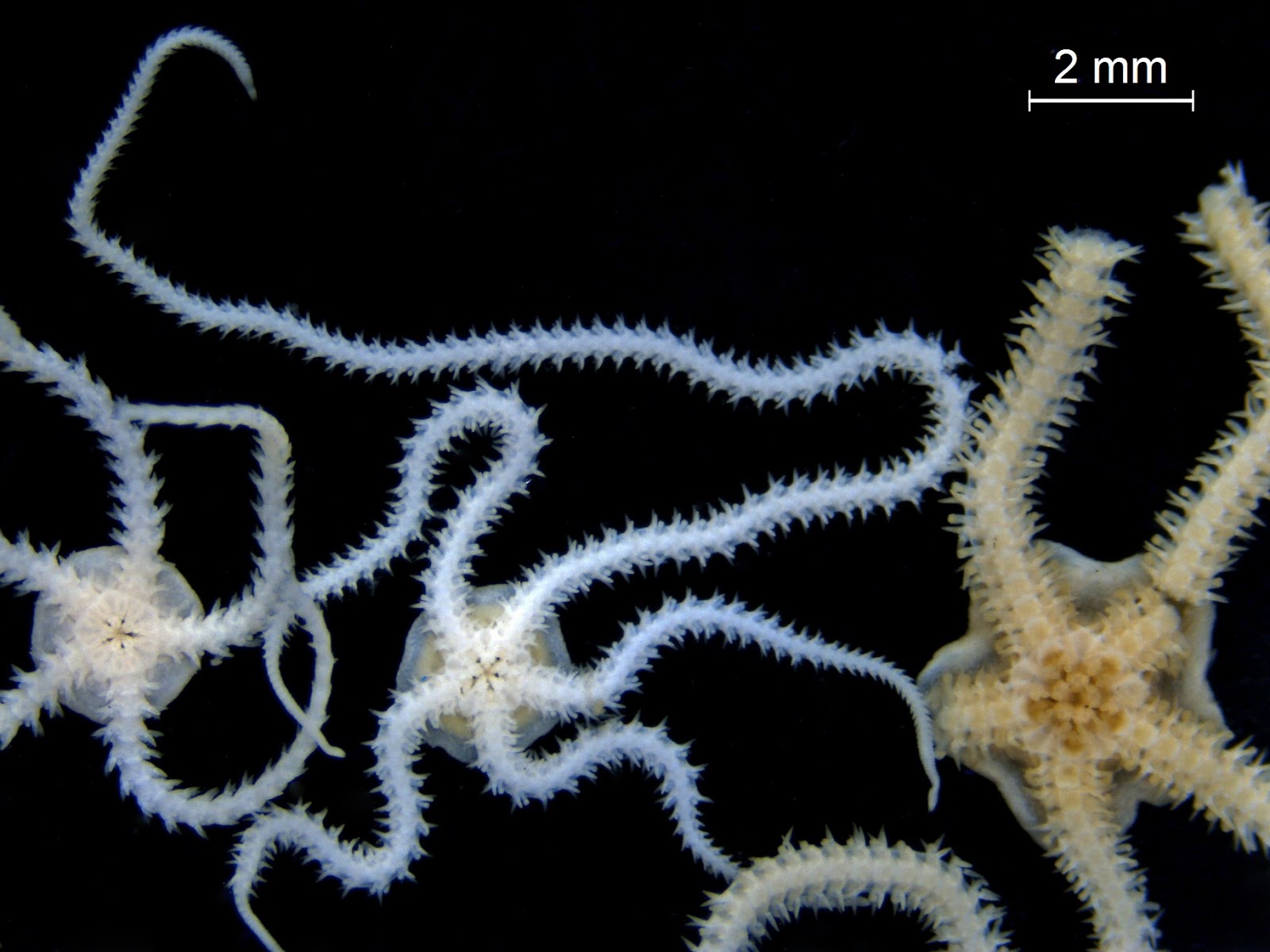The image in landscape orientation reveals a highly detailed, microscopic view of three starfish-like sea creatures set against an entirely jet-black background. In the top-right corner, white text indicates a scale of "2mm" for reference. The creatures range in color from tan to varying shades of light blue and white. The largest, positioned centrally, is tan and noticeably thicker, with five shorter, more robust legs—one of which appears to be missing. To its left, a slightly smaller creature in light blue displays five long, spindly legs that twirl out from its center. Another similar light blue specimen lies next to it, also featuring remarkably elongated, thin legs. All legs extend in a radial pattern from their central bodies, which display a distinct central opening, likely indicative of their mouths. The detailed image highlights the intricate textures and varying tentacle lengths of these fascinating marine creatures.